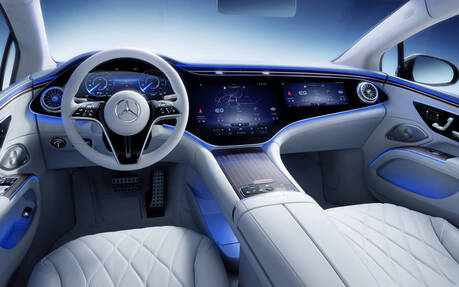The image captures the interior of a futuristic Mercedes-Benz, taken from the perspective of someone sitting in the back seat and looking forward. The dashboard is packed with advanced digital interfaces, featuring prominent, iPad-like screens concentrated in the center and passenger areas, likely for controlling entertainment options, climate settings, and other functionalities. The driver's side is dominated by a modern, high-tech steering wheel adorned with a large, unmistakable Mercedes-Benz logo, flanked by digital round dials acting as a speedometer and tachometer. The interior is elegantly designed with white, tufted bucket seats and a matching center console and pillars, contrasted by a dark, complex dash highlighted with blue LED lighting, which also illuminates the door handles and speakers. The overall color theme balances between white, light gray, and dark tones, creating a sleek and ultra-modern atmosphere.